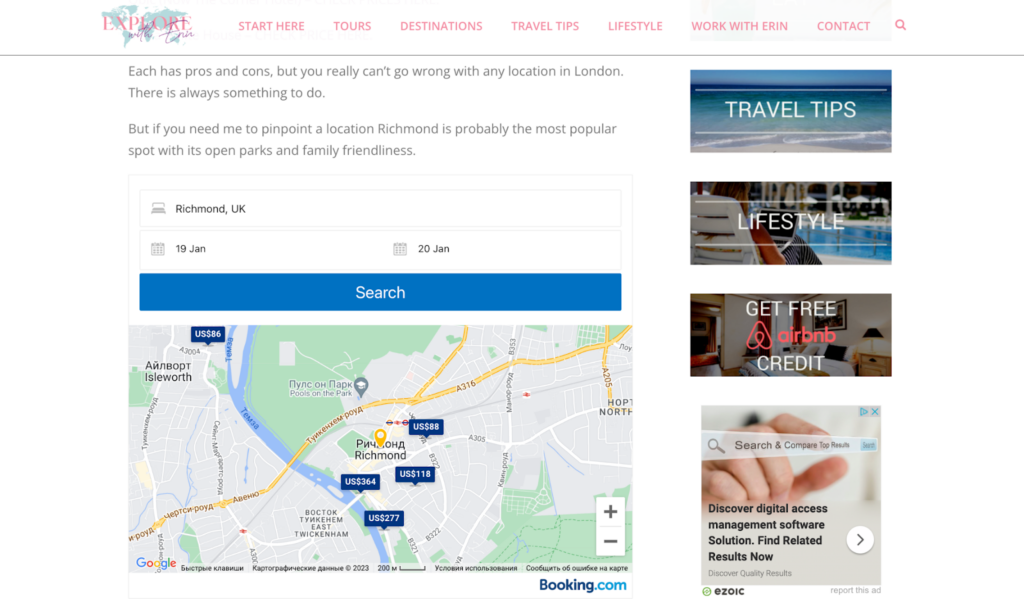**Website Screenshot of "Explore with Erin" - Travel Recommendations for London**

The image is a horizontal screenshot from a website, displayed against an indistinct white background, akin to a computer screen. At the top-left corner, the branding "Explore with Erin" is prominently visible, accompanied by a small, teal-colored icon of the continents. Below the branding are several navigation options highlighted in a soft pink color: "Start Here," "Tours," "Destinations," "Travel Tips," "Lifestyle," "Work with Erin," and "Contact." Notably, the "Work with Erin" and "Contact" options are emphasized with a subtle gray bar.

The main content of the image discusses travel destinations within London, highlighting that "each has its pros and cons" and suggesting that "you can't really go wrong" with any location. Specifically, it recommends Richmond as a popular spot due to its open parks and family-friendly environment.

Following this, two calendar dates are displayed, the 19th and 20th of January, denoting potential travel dates to Richmond, UK. Adjacent to the dates is a clickable blue search bar button.

Further down, a map, presumably from booking.com, is shown, pinpointing locations and travel options in Richmond. On the right-hand side, a vertical column lists additional navigation and search features: "Travel Tips," "Lifestyle," "Get Free Airbnb Credit," and a "Search and Compare Top Results" option.

This comprehensive layout provides a user-friendly interface for exploring travel advice and booking options with Erin's guidance, making it easy to plan a trip to Richmond, London.